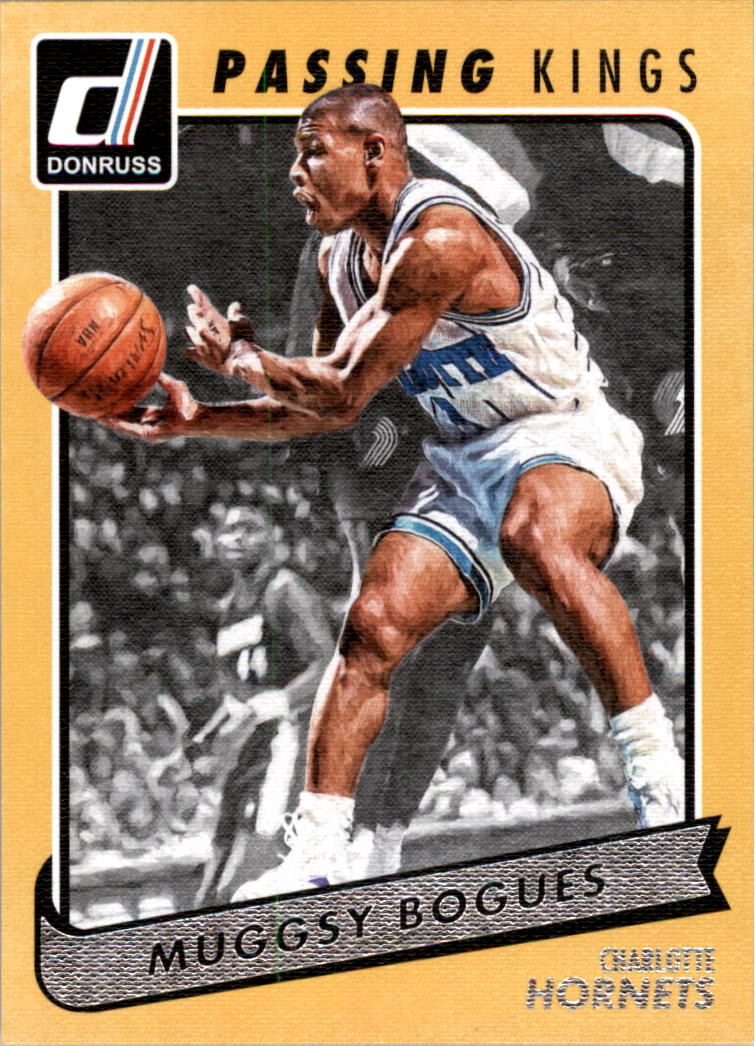This image is a professionally rendered action shot of a basketball trading card, likely from the Donruss brand, known for its "Passing Kings" series. The background is a yellow-tinged peach color, prominently featuring an African-American player identified as Muggsy Bogues from the Charlotte Hornets. Bogues is depicted mid-action, seemingly about to catch an orange and black basketball marked with "NBA." He wears a white, sleeveless jersey with "Charlotte" written in blue lettering across the chest, paired with white shorts featuring blue trim, white socks, and white sneakers. His mouth is open, possibly shouting or calling a play. The card also includes a vivid depiction of the audience and another player in the background, this player donned in a dark uniform with white lettering and the number 44. There is a "D" logo in red, white, and blue in the corner, signifying Donruss, with "Donruss" written beside it. At the bottom of the card, it distinctly states "Muggsy Bogues," with "Charlotte Hornets" beneath it.